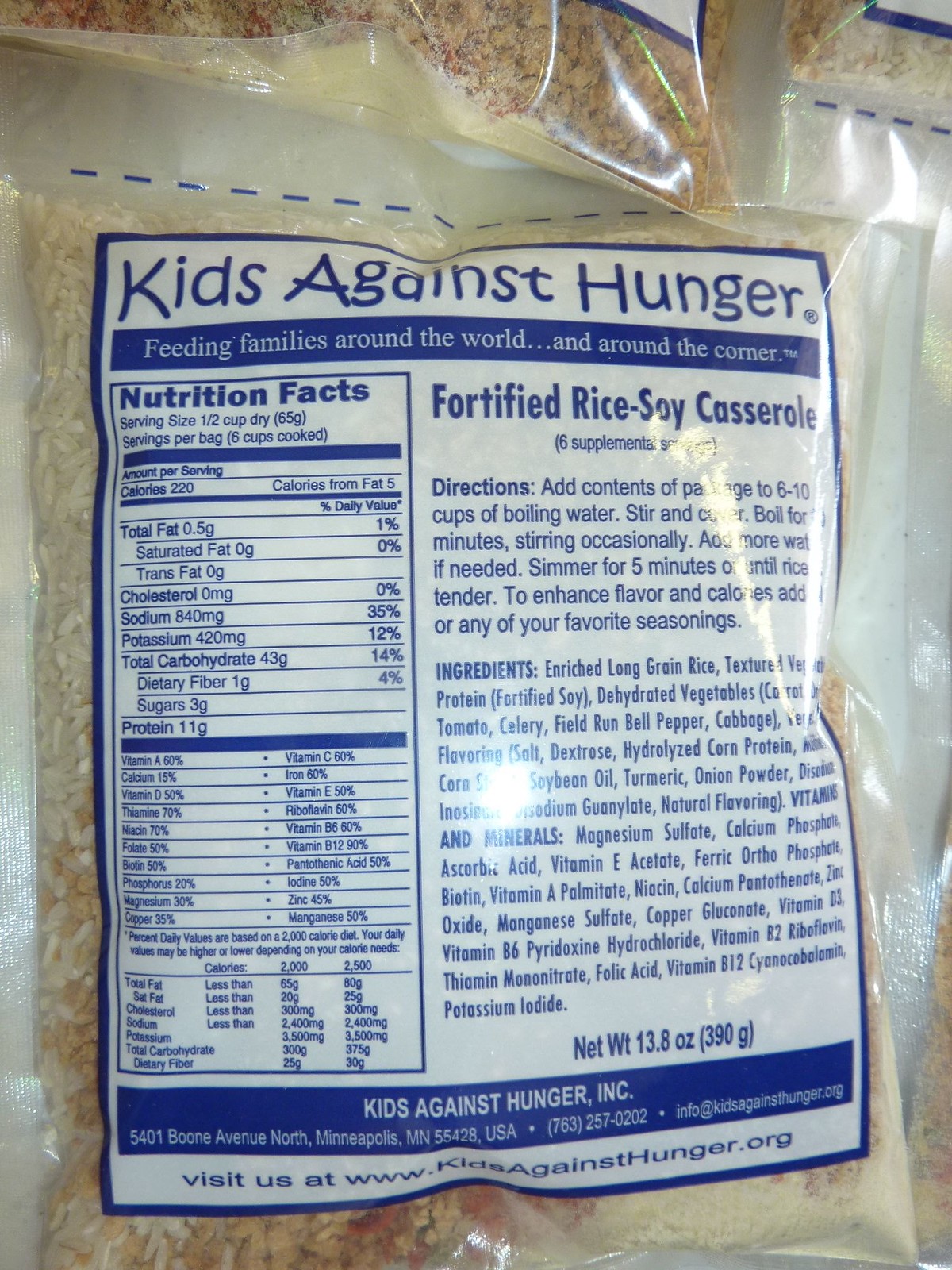The image depicts the back of a clear plastic food package containing rice mixed with dried spices and vegetables. The packaging features prominent blue text on a white background, including the logo "Kids Against Hunger: Feeding Families Around the World and Around the Corner." The bag holds 13.8 ounces (390 grams) of fortified rice soy casserole, providing six supplemental servings. You can see individual rice grains along with red and brown specks through the clear packaging. The cooking instructions advise adding the package’s contents to 6 to 10 cups of boiling water, stirring, then covering and boiling for an unspecified duration. Afterward, simmer for five minutes until the rice is tender, with suggestions to enhance flavor and calories by adding meat or favorite seasonings. The packaging also lists the nutritional information and ingredients, and it includes contact details and a website: www.kidsagainsthunger.org.